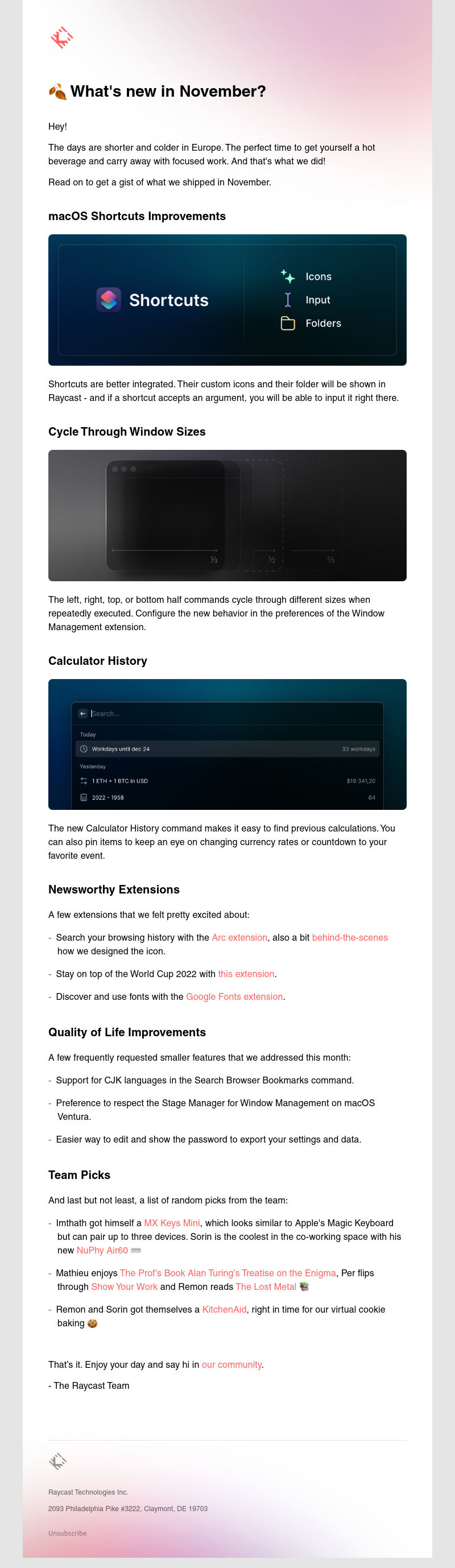"What's New in November: As the days in Europe grow shorter and colder, it's the perfect time to cozy up with a hot beverage and dive into some focused work. And that's exactly what we've been up to. This month, we've shipped several exciting updates:

- **macOS Shortcuts Improvements**: Shortcuts are now better integrated into Raycast. Custom icons and folders for your shortcuts are now displayed, and if a shortcut accepts an argument, you can input it directly within Raycast.
- **Cycle Through Window Sizes**: Execute commands to cycle through different window sizes for the left, right, top, or bottom areas of your screen. Configure these new behaviors in the preferences of the Window Management extension.
- **Newsworthy Extensions and Quality of Life Improvements**: We've also added several noteworthy extensions and enhancements to improve your overall experience.
- **Team Picks**: Discover our curated selections for the month. 

Enjoy your day, and don’t forget to say hi in our community forum. - The Raycast Team"